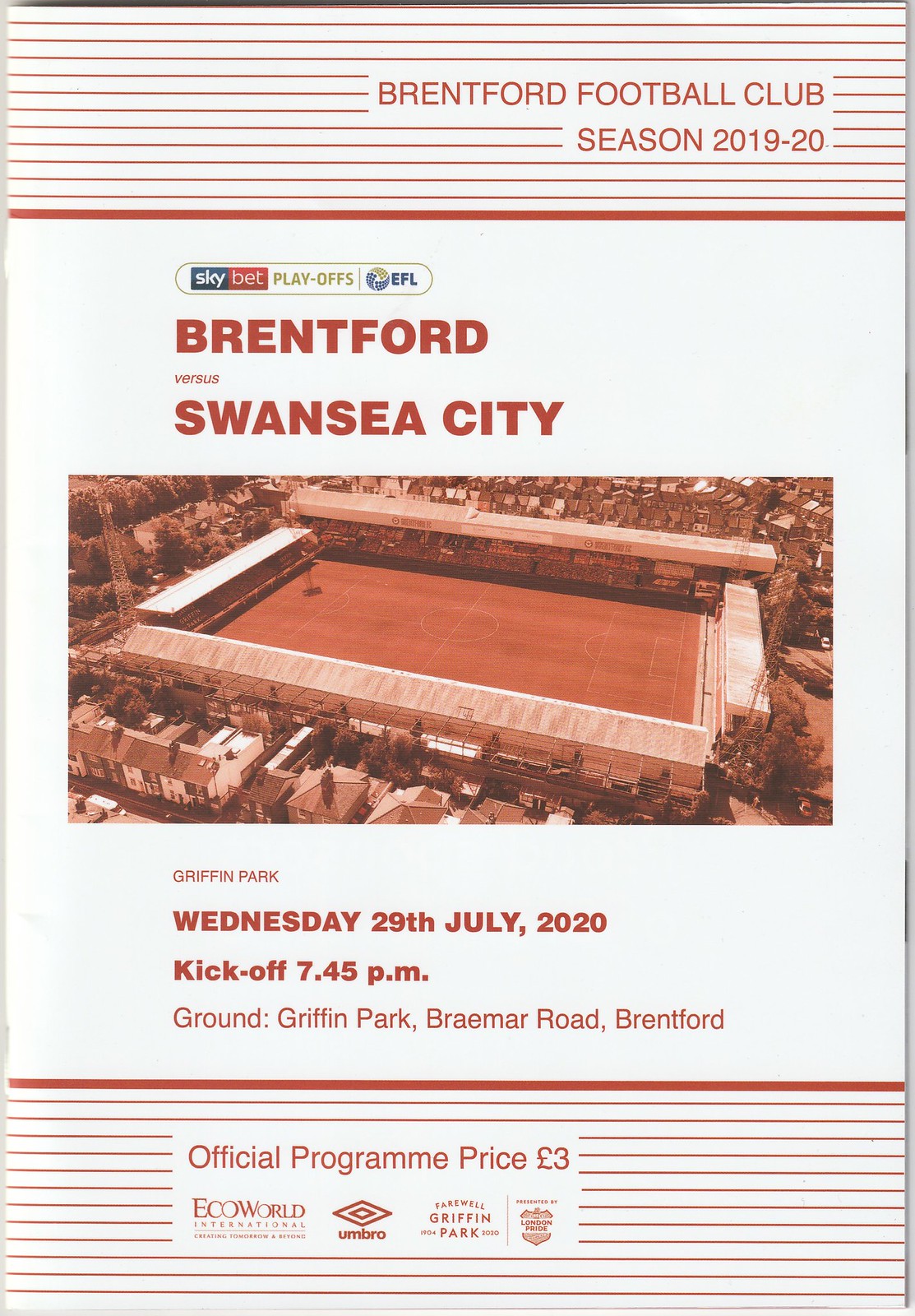This image is a detailed cover of the official game day program for Brentford Football Club’s match against Swansea City during the Sky Bet Playoffs EFL Season 2019-20. The cover features a distinct design with red stripes at the top and bottom of the page. The top section includes the red text "Brentford Football Club Season 2019-20" prominently displayed against a white background, accompanied by a small logo indicating the Sky Bet Playoffs EFL. Below this, an aerial sepia-toned photograph of Griffin Park showcases the stadium along with the surrounding community buildings. The text below the image details the event specifics: "Griffin Park, Wednesday, 29th July 2020, Kickoff 7.45pm, Ground Griffin Park, Braemar Road, Brentford." The lower section includes a white rectangle bordered by red stripes, stating "Official Program Price £3." Additional sponsorship logos are displayed in this section, alongside the phrases "Eco World International Creating Tomorrow and Beyond" and "Farewell Griffin Park presented by London Pride."